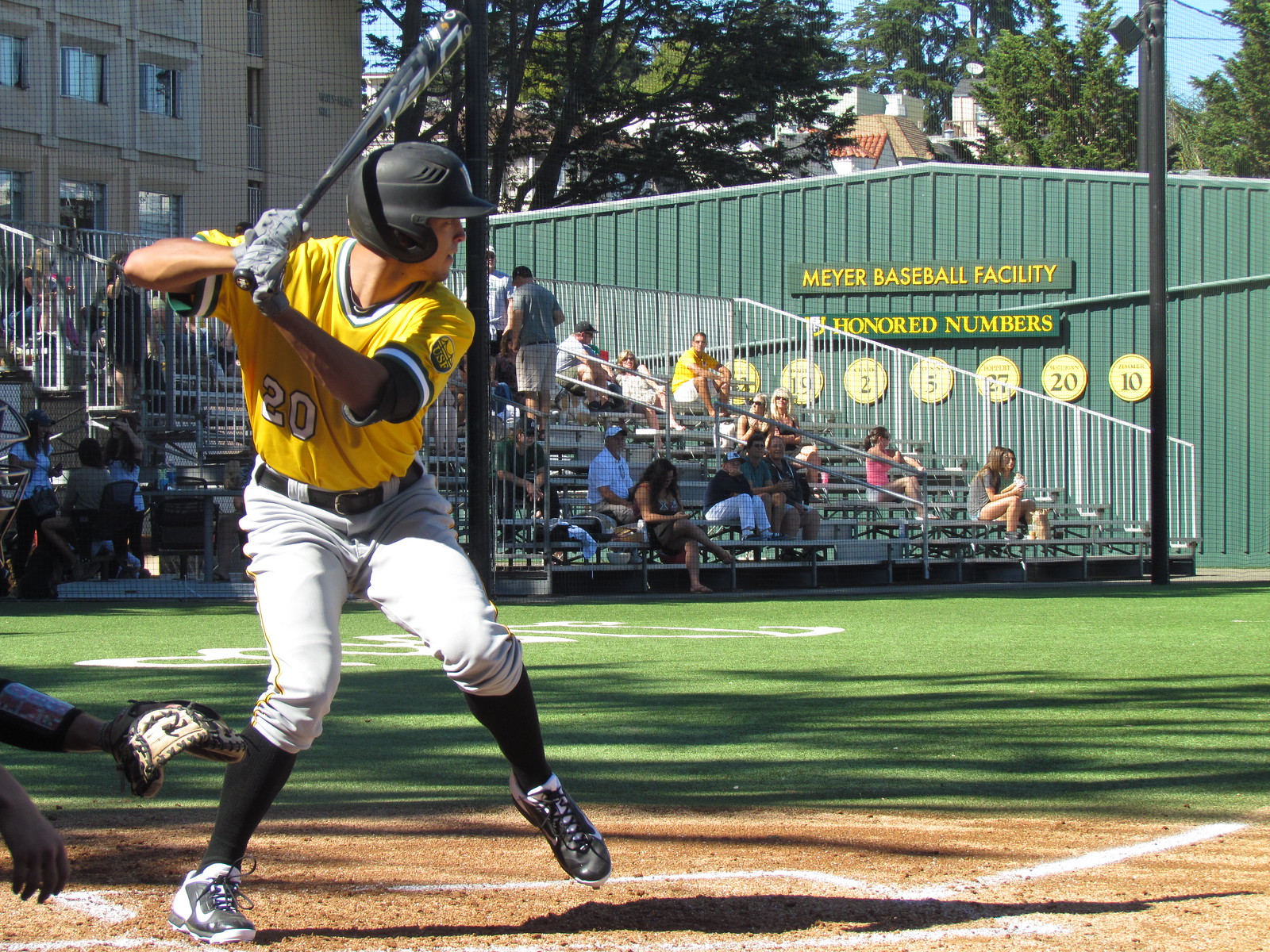This vividly detailed image captures a moment in a baseball game, featuring a young man poised to swing his bat. The scene is brightly lit, suggesting a clear, sunny day. The player, dressed in a yellow v-neck uniform with the number 20 and black and white accents, is in profile, revealing his determined expression. His gray pants are adorned with a gold stripe down the sides, and he completes his outfit with black socks and black cleats bearing a white Nike symbol. His gray baseball gloves grip a black metal bat, and a protective helmet sits snugly on his head. 

He stands on the left side of the image, ready in the batter's box. Behind him, the catcher’s extended, gloved left hand and part of his face are just visible. The well-manicured field extends below, with bright green turf transitioning to a mix of brown and light brown sand nearer the bottom.

In the distance, silver bleachers host a small crowd, dressed in a variety of warm-weather attire, from short sleeves to tank tops and shorts to jeans. Their appearances vary widely, with different hair colors and styles and a mix of hats and sunglasses. Behind these spectators, a green building prominently displays "Meyer Baseball Facility" in yellow lettering. The structure also features a sign labeled "Honored Numbers," with some visible numbers including 19, 2, 5, 27, 20, and 10, hinting at the facility's storied history, possibly linked to a minor league or collegiate team.

To the left, more buildings, which may be residential or educational, peek into view, along with some trees, adding depth to the scene. The field is equipped for night games, evidenced by the presence of lighting poles and amplifiers. This image, likely about 6 by 7 inches, immerses the viewer in the atmosphere of a lively, perhaps community-level, baseball game.